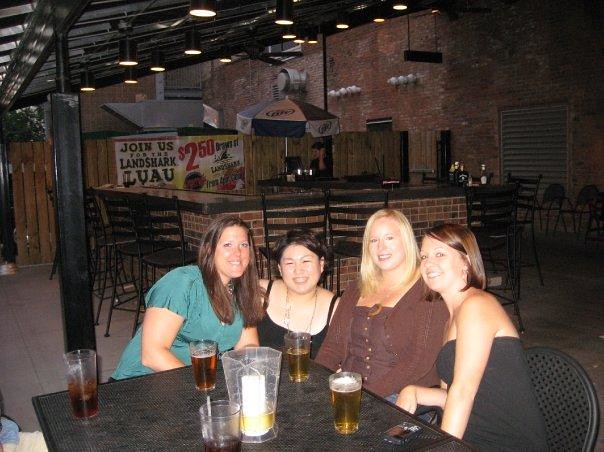In this detailed image, four women, likely friends in their late twenties or early thirties, are seated around a black table with black bar stools or chairs in a bar or restaurant with a cozy, perhaps outdoor seating area. The environment features warm, red brick walls and a black countertop bar. There is a hint of outdoor elements like trees visible through what could be an awning-type roof. Two women have brown hair—one long and one short—while another has long blonde hair, and the fourth has short dark brown hair. They are all smiling and leaning close together, creating a sense of camaraderie and fun. On their table, there is a pitcher of beer and four glasses, though one glass appears to contain a drink with ice, suggesting it might be something other than beer. The ambiance is further detailed with signs behind the bar, one advertising a "Landshark LUAU" and another promoting a $2.50 special. The black countertop and bar stools add a modern touch to the rustic brick surroundings, and there might be kitchen equipment in the background, hinting it could also serve food.